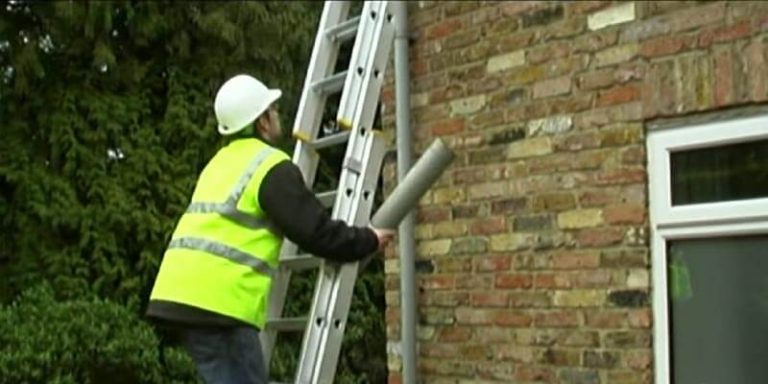In this image, a worker is captured mid-climb on a metal ladder propped against a brick building, potentially a home. He is clad in a bright fluorescent yellow reflective safety vest over a black long-sleeve shirt, coupled with jeans and a white hard hat. The worker, positioned a few rungs up the ladder, holds a large silver pipe or tube in his right hand, suggesting he might be engaged in construction or repair work like fixing a gutter or a drain. The scene is set outdoors, in what appears to be a rural area with a dense thicket of trees surrounding the building, visible on the left side of the image. The brick structure itself looks somewhat old, featuring a white-framed window at the far right edge of the photo. The day seems overcast, lending a slightly blurry quality to the background, which includes more trees and a central pipe running down the building façade.